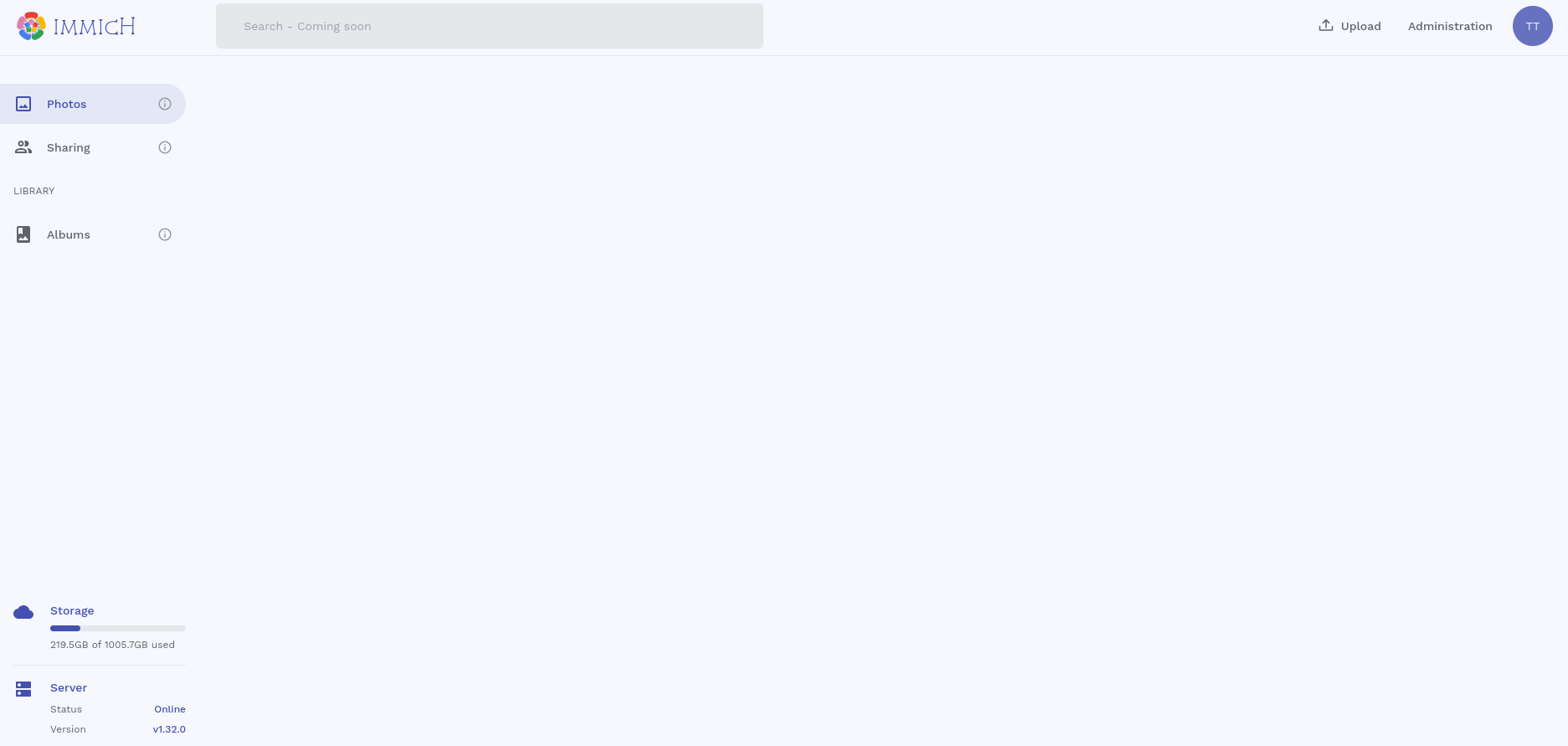The image depicts a screenshot from a website with a light blue background. At the top of the screen, there is an emblem resembling a flower with six petals in different colors: red, golden yellow, green, blue, and maroon pink. Next to the flower, in capital letters, it reads "I M M I C H."

Below this, there is a gray search bar with the text "search coming soon." On the left side of the screen, a navigation tab labeled "photos" in blue text includes an information icon (a small circle with an "i" inside).

Further down, there is a graphic illustration showing two stylized head-and-shoulder figures with the text "sharing" and another information icon next to it. Below this, options for "library" and "albums" each feature a similar information icon.

At the bottom of the left side, there is an icon of a cloud labeled "storage," showing the storage usage as "2.19.5 GB of 1,005.7 GB used." The text "server status version outline B 1.3 2.0" appears at the bottom.